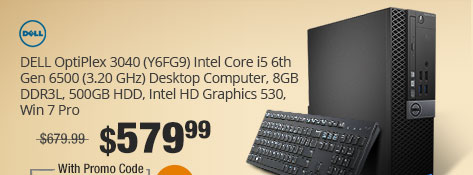The image is a partially visible screenshot of an advertisement for a Dell computer, formatted as a horizontal rectangle. The background has a gradient, starting as a darker beige color in the left corner and gradually lightening towards the right. In the top left corner, the familiar blue Dell logo is present, featuring the word "Dell" inside a blue circle. 

Beneath the logo, detailed specifications for the Dell Optiplex 3040 are listed:

- Model Number: (Y6FG9)
- Processor: Intel Core i5 6th Generation 6500, clocked at 3.20 GHz
- Type: Desktop Computer
- Memory: 8 GB DDR3L
- Storage: 500 GB HDD
- Graphics: Intel HD Graphics 530
- Operating System: Windows 7 Pro

The original price of $679.99 is crossed out, highlighting a sale price of $579.99 in large black type. Below the sale price, there's a mention of an additional discount available with a promo code. 

The visual elements include images of the Dell computer itself and an accompanying black keyboard, positioned prominently within the ad.